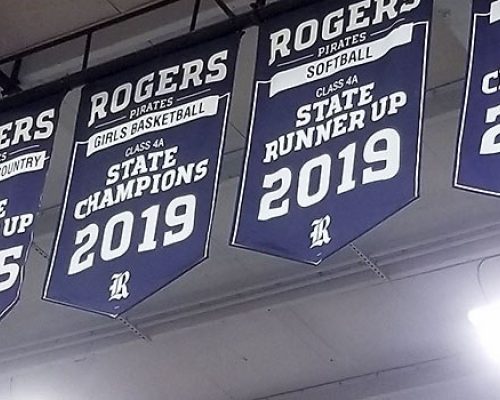This landscape photograph, taken in color, captures banners hanging from the roof of a sports stadium, likely taken by someone seated in the bleachers. The image is aimed at the top of the arena, showcasing the achievements of the Rogers Pirates teams, prominently featuring two entirely visible blue banners with white lettering. The first banner reads, “Rogers Pirates Girls Basketball Class 4A State Champions 2019”, and the second one states, “Rogers Pirates Softball Class 4A State Runner-Up 2019”. Each banner features a distinctive "R" logo at the bottom, possibly representing the Rogers Pirates' emblem. Additionally, there are glimpses of two more banners partially visible at the edges of the frame. The backdrop reveals the stadium's ceiling structure with its scaffolding and lighting, emphasizing the setting within a sports arena.